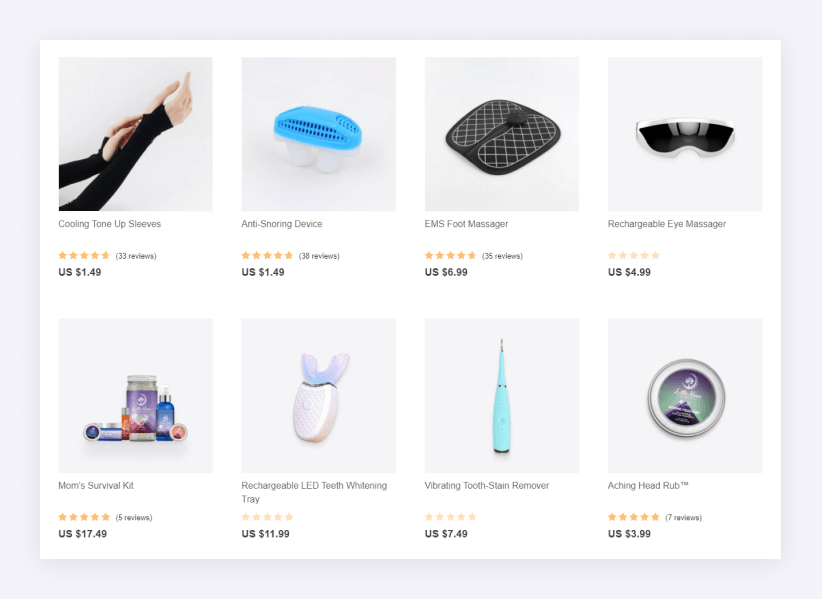The image is a screenshot showcasing an online shopping interface where a user is browsing eight distinct products. The background of the screen features a gray hue, providing contrast to the central white area where the products are displayed. Each product image is set against a white background with a subtle gray tint to make them stand out. The products are arranged in two rows, with four items in each row.

In the first row:
1. The first product on the left is "Cooling Tone-Up Sleeves," priced at $1.49.
2. Next is an "Anti-Snoring Device," also priced at $1.49.
3. The third item is an "EMS Foot Massager," available for $6.99.
4. The final product in the first row is a "Rechargeable Eye Massager," listed at $4.99.

In the second row:
1. The first product on the left is a "Mom's Survival Kit," priced at $17.49.
2. Adjacent to it is a "Rechargeable LED Teeth Whitening Tray," for $11.99.
3. The third item is a "Vibrating Tool Stain Remover," which costs $7.49.
4. The last product is an "Achy Hand Rub," priced at $3.99.

Each product display includes a rating system indicated by stars.